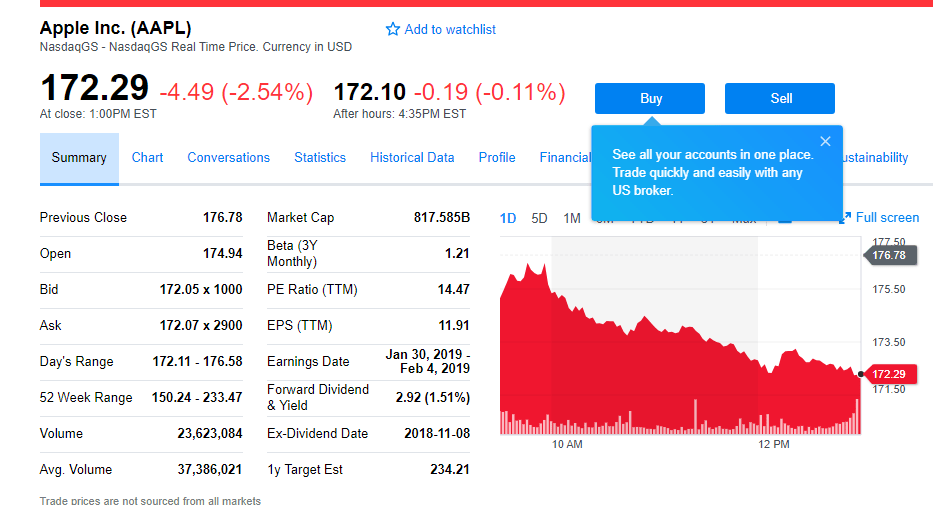Caption: 

This image presents a detailed stock analysis from Apple Inc. (AAPL), listed on NASDAQ GS in real-time with prices displayed in USD. A prominent graph on the right showcases the stock's performance, marked in bold red lines that resemble an EKG pattern. These red lines depict the changes in stock price, rising and falling over the trading hours. Directly beneath the red lines, white column-like bars indicate volume trades, mirroring the ups and downs of the stock.

A closer look at the time markers along the bottom reveals significant activity between 10 AM and 12 PM, where the stock price peaks at 10 AM and then drops considerably by 12 PM. The chart is set to display a one-day overview, as indicated by the highlighted blue section labeled "one day." The current closing price is shown as $172.29 at 1 PM, alongside various volume ratio metrics and other related financial data.